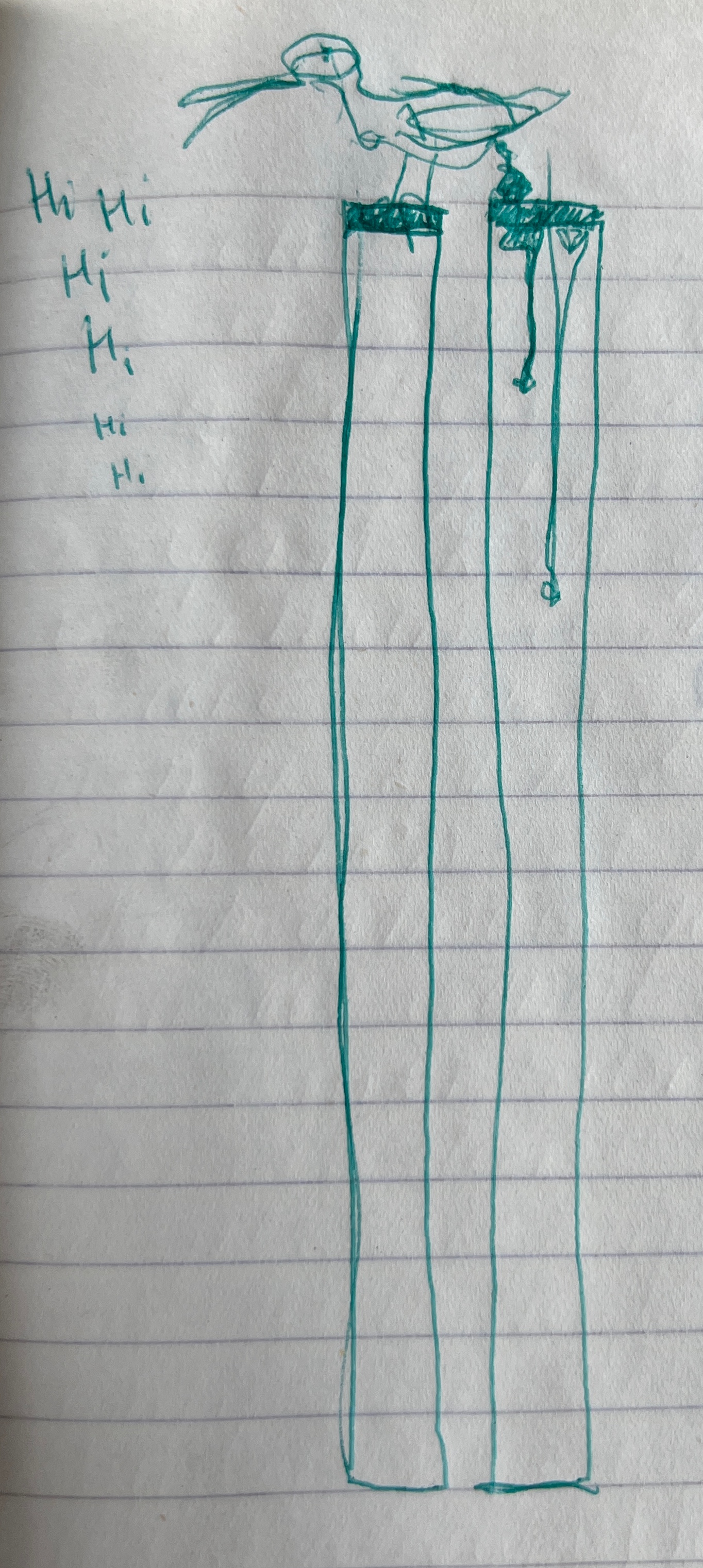The image depicts a notebook with lined pages, prominently illustrated with a drawing. At the top of the page, a bird, rendered primarily in green ink, is depicted with a large beak and an elongated body. The bird is perched on two extraordinarily tall towers, straddling both with each foot placed on a different tower. The scene becomes more provocative as the bird is shown defecating on the right tower, with liquid visibly cascading down the side. The drawing, while crude and possibly innocent in intention, evokes a strong and potentially controversial resemblance to the Twin Towers, prompting an intense reaction from viewers.